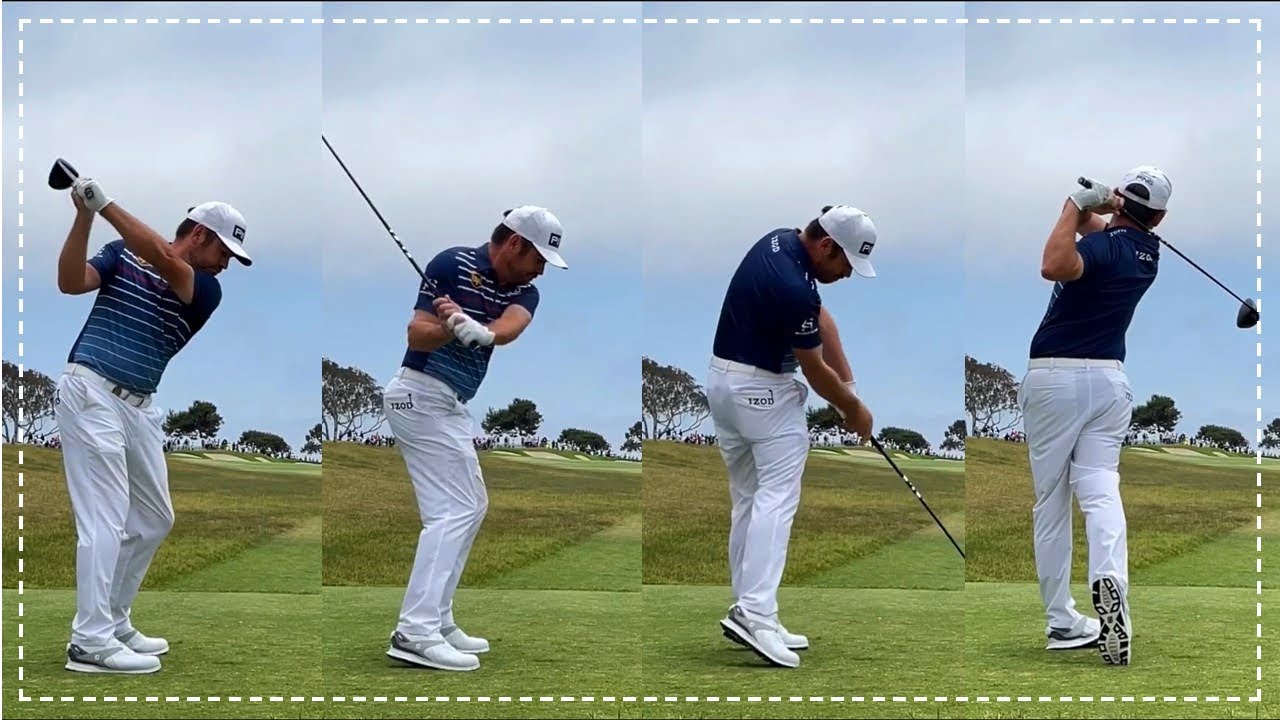The image depicts a man on a golf course, shown in a sequence of four distinct frames that capture the various stages of his golf swing, arranged from left to right. The man is dressed in golfing attire which includes a blue shirt with white stripes, white pants, white shoes with gray and black treads visible on the sole, and a white belt. He also wears a white cap featuring some unreadable lettering. Notably, the clothing brand "IZOD" is printed on the back of both his shirt and pants. He sports a white glove on his left hand and is holding a black driver golf club. The background showcases a clear sky with some clouds, and trees lining the horizon, set against varying shades of well-manicured green grass. The border of the image is adorned with a white dotted line, framing the four sequential photos that intricately detail the phases of his swing, from the wind-up, mid-swing, contact, to the final follow-through stance.